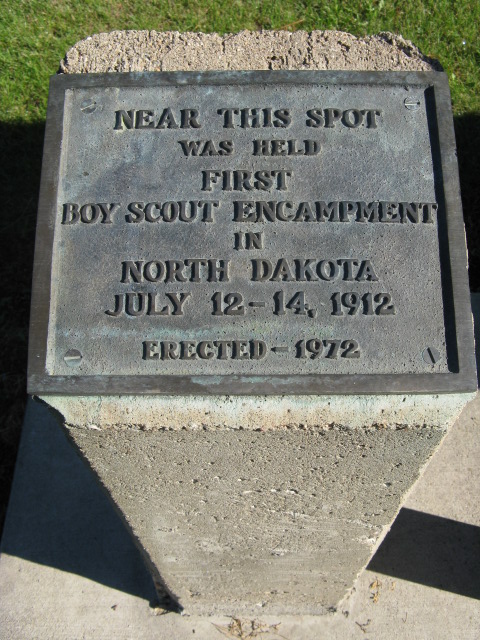This image features a memorial dedicated to the first Boy Scout encampment in North Dakota, which took place from July 12th to 14th, 1912. Erected in 1972, the memorial consists of a beige-colored concrete block with noticeable cracks, indicating its age. The block supports a metal plaque, likely made of brass or copper due to its greenish hues from weathering. The plaque itself is grey with a beveled edge and has raised text. The inscription reads: "Near this spot was held first Boy Scout encampment in North Dakota, July 12–14, 1912. Erected, 1972." This set-up is situated on a flat concrete base, surrounded by neatly cut green grass. The scene is well-lit by sunlight, which casts distinct shadows of the memorial on the ground, emphasizing its shape and structure. Four screws, one at each corner, secure the plaque in place, completing this historical marker commemorating an important event in Boy Scout history.